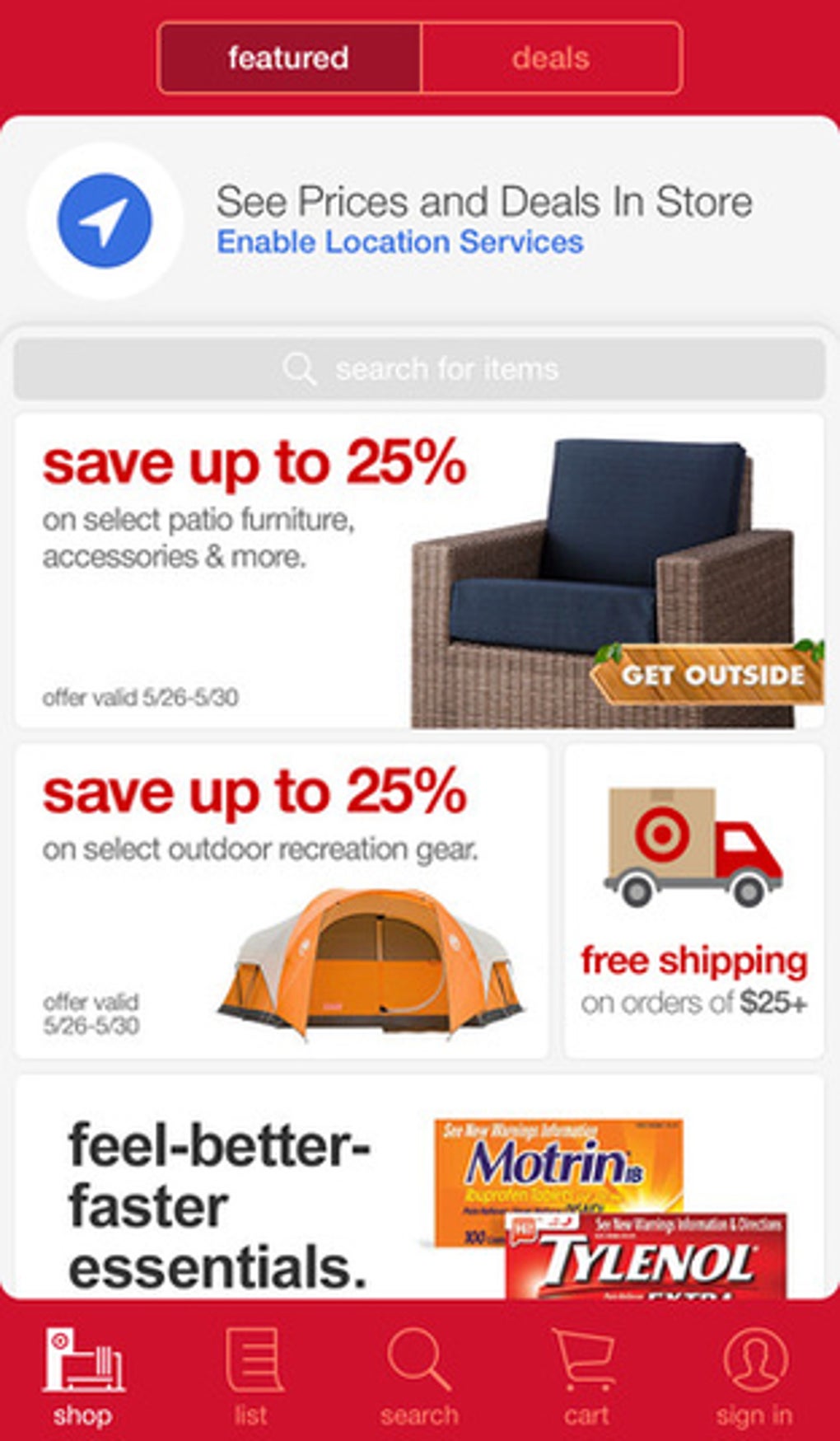Detailed Caption: 

The image shows a screenshot from a shopping session on Target's website, likely taken from a phone, laptop, or desktop. At the very top of the page, there's a prominent red header featuring two distinct sections. One is a long search box, and to its left, there's a darker red box with the word "Featured" in white. Adjacent to it is the word "Deals," displayed in a grayish hue.

Beneath this header, the background shifts to white. On the left side, there's a solid blue circle with a diagonal right-pointing arrow. Beside this icon is the text "See prices and deals in store," written in large gray font. Directly below this, in blue text, it says "Enable location services." Following this is a smaller gray search box labeled "Search for items."

Further down the page, on the left, red text in lowercase reads "save up to 25% on select," and below it, in a smaller gray font, "on select patio furniture, accessories, and more." To the right of this text, there’s a diagonal view of an outdoor chair with a blue crochet cushion, featuring a brown wicker design.

Below this section, the text "save up to 25%" appears again in red, referring to "select outdoor recreation gear." Adjacent to this, on the right, is a side view of an animated Target truck with a bullseye logo. Below the truck, it states "free shipping" in red, with "on orders of $25 plus" in gray underneath.

To the left, there’s a front view of a camping tent; its top and sides are orange with some white patches on the edges. Below this, in bold black font, it reads "feel-better-faster essentials." Next to this text, there’s an image of an orange box with blue lettering that says "Motrin." Below the Motrin box, there’s a red box with white text that reads "Tylenol."

At the bottom of the image, there is a red strip with multiple icons and labels. From left to right, it includes a shop icon, a list icon, a magnifying glass labeled "research," a cart icon, and a circle with a person’s silhouette labeled "sign in."